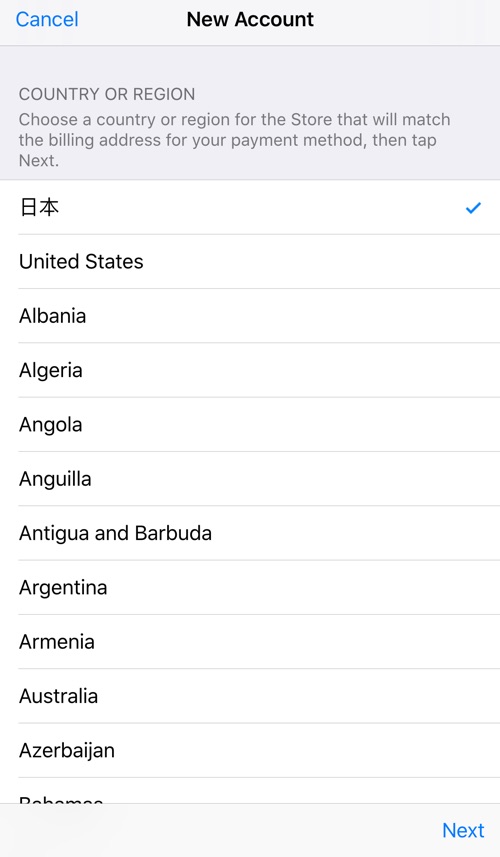The image showcases a user interface for setting up a new account, displayed within a vertically oriented rectangular section. At the very top-left corner, there's a blue "Cancel" button. Centered at the top of the section is the title "New Account" in black text.

Beneath the title, a shaded box contains a three-line instruction. The instruction begins with "Country or Region" followed by a brief white space. The full text of the instruction reads, "Choose a country or region for the store that will match the billing address for your payment method, then tap Next." Notably, the "C" in "Choose," the "S" in "Store," and the "N" in "Next" are capitalized, despite the sentence case structure.

Below this shaded instruction box, the interface returns to a white background. Here, a dropdown list of countries is presented on lined white paper. The list begins with a country represented by two Chinese symbols, marked with a blue checkmark on the right. Following the foreign symbols, several countries are listed in alphabetical order: United States, Albania, Algeria, Angola, Antigua and Barbuda, Argentina, Armenia, Australia, Azerbaijan, and partially visible, Bahamas.

At the bottom of the screen, there is a gray section featuring a blue "Next" button, indicating the user can proceed after making their country selection.